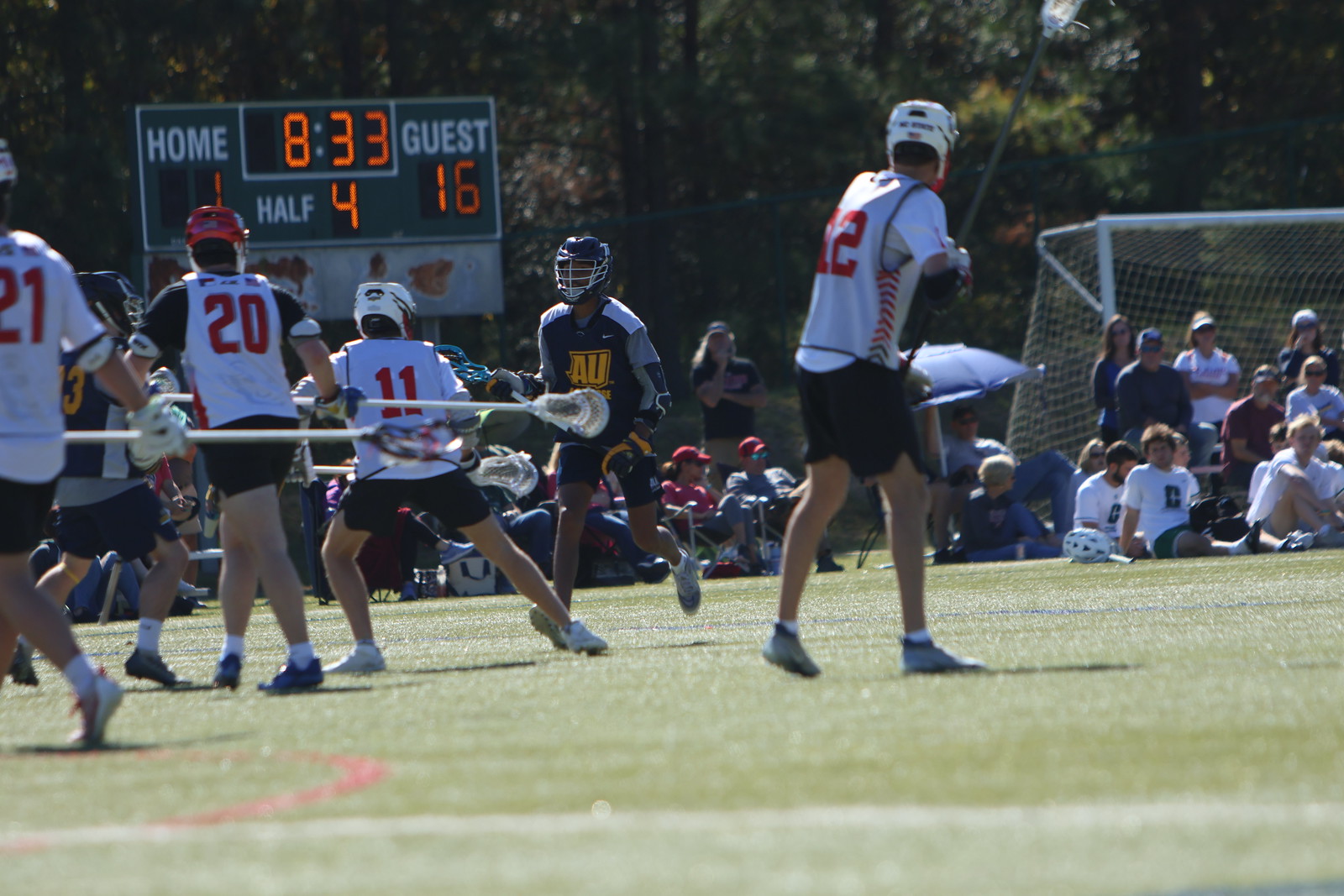The photograph captures an intense lacrosse game under a sunny sky, likely at high noon given the short shadows. The scoreboard dominates the upper left corner, displaying a lopsided score of 1 for the home team and 16 for the guests, with 8 minutes and 33 seconds left in the fourth period. The game takes place on a verdant field marked for lacrosse, with four players in white jerseys – numbered 21, 20, 11, and 22 – in various stages of play. A fifth player, in a black jersey with "AU" in gold, stands out prominently. Despite the clear mismatch in scores, the spectators, some seated on the grass or in lawn chairs along the sidelines, create a vibrant atmosphere. The field is bordered by trees, adding a scenic backdrop to the energetic game. The goal net is positioned on the right side of the image, with some spectators sitting intriguingly close but off to the side. The players hold lacrosse sticks, intensifying the action and the sport’s dynamic appeal. This picture embodies the spirit and competitive nature of lacrosse, amidst engaged fans and a picturesque setting.